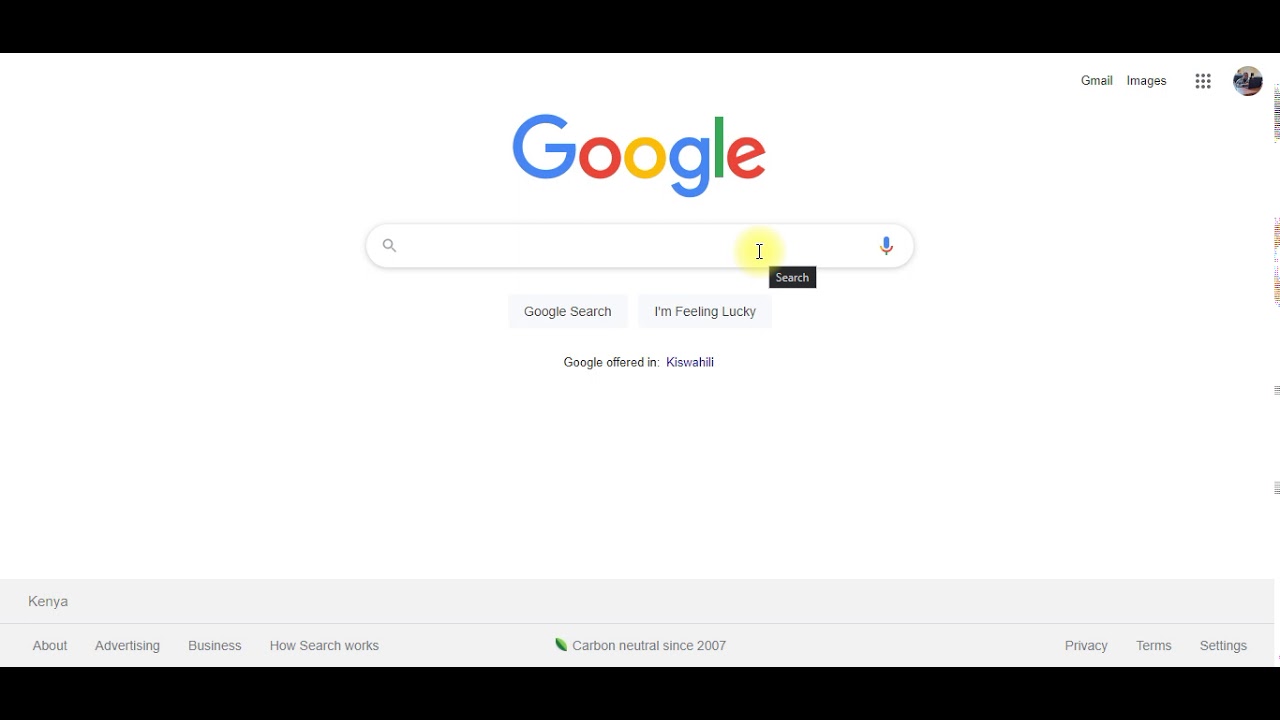The image depicts a widescreen view with horizontal black bars at the top and bottom, reminiscent of a cinematic aspect ratio. At the center of the image lies the main Google search page, set against a clean, white background. 

In the top right corner, there are links labeled "Gmail" and "Images," along with a grid icon comprising three rows of three dots and a user profile picture. 

Dominating the center is the iconic Google logo, with the letters "G" in blue, "o" in red, "o" in yellow, "g" in blue, "l" in green, and "e" in red. Below the logo is a search bar, currently active with a cursor blinking and highlighted by a subtle yellow glow. Inside the search bar is the prompt "Search."

Beneath the search bar are two buttons: one labeled "Google Search" and another labeled "I'm Feeling Lucky." Following these, there is a phrase stating "Google offered in Kiswahili."

At the very bottom of the screen, a gray footer bar spans the width of the page. On the left side of this bar, "Kenya" is noted. Further left-aligned items include links labeled "About," "Advertising," "Business," and "How Search Works." Centrally positioned within the footer is the statement "Carbon neutral since 2007," accompanied by a small green leaf icon. The right side of the bar features links labeled "Privacy," "Terms," and "Settings."

The overall aesthetic is minimalistic and clean, adhering to Google's traditional style, with the multicolor logo providing a burst of familiar, comforting colors against the white background.